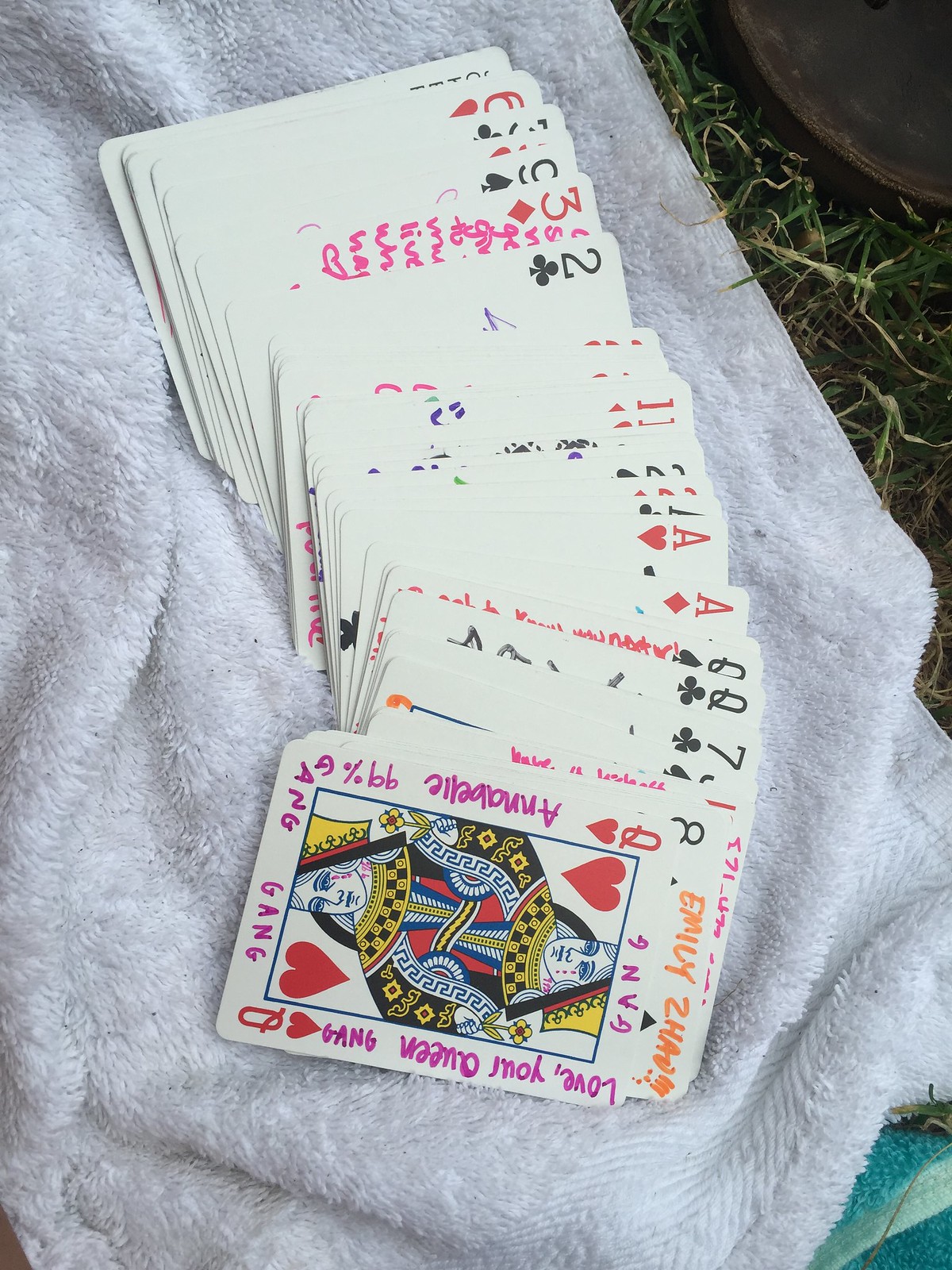The image captures a deck of playing cards fanned vertically atop a pristine white towel, which occupies the majority of the left-hand side of the photograph. The towel is laid on a grassy surface, with a hint of greenery visible in the upper right corner. Adding to the outdoor ambiance, an indistinguishable brown object, potentially an outdoor seat, is also visible in the upper right section. In the bottom right corner, a sliver of another towel, this one blue, peeks into the frame.

The white-background cards exhibit a traditional design, and are marked with unique handwritten phrases in marker around their outer borders. The Queen of Hearts, positioned at the top of the deck, features intriguing annotations such as "Love your Queen," "Gang," "Emily Zhao Gang," "Annabelle," and "99% Gang Gang." These playful inscriptions suggest the deck belongs to a younger individual, possibly an Asian college student, who has personalized the cards for amusement or as a creative project.